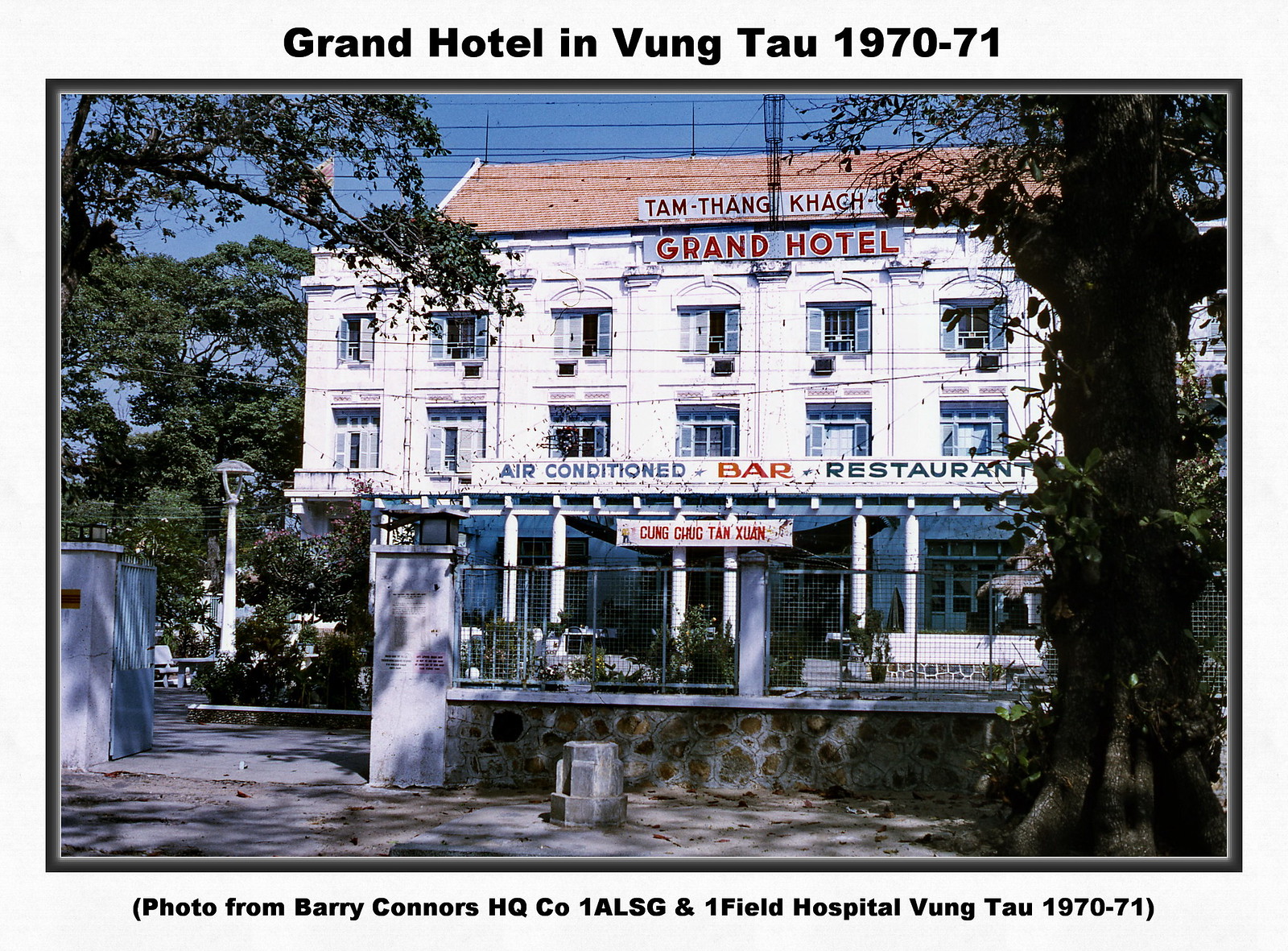This detailed image, credited to Barry Connors HQ, CO1ALSG, in Onefield Hospital of Vung Tau, 1970-1971, showcases the Grand Hotel in Vung Tau during the years 1970-71. The older, multi-story building boasts a white exterior complemented by a light reddish-tan roof. Prominent bright blue moldings frame the windows, which are noted for their uniform blue shutters. Nestled between trees on either side, the hotel stands behind a small stone wall and a metal fence. A red-lettered sign prominently announces "Grand Hotel," alongside another sign advertising an "Air Conditioned Bar and Restaurant.” Additional text on the building, "Tam Thang Kok Grand Hotel” can also be seen, alongside another sign with text that is difficult to pronounce, likely in a local language. Displayed on a white-bordered sign at the bottom, black text credits the photo to Barry Connors of the HQ CO1ALSG and One Field Hospital, Vung Tau, 1970-71.